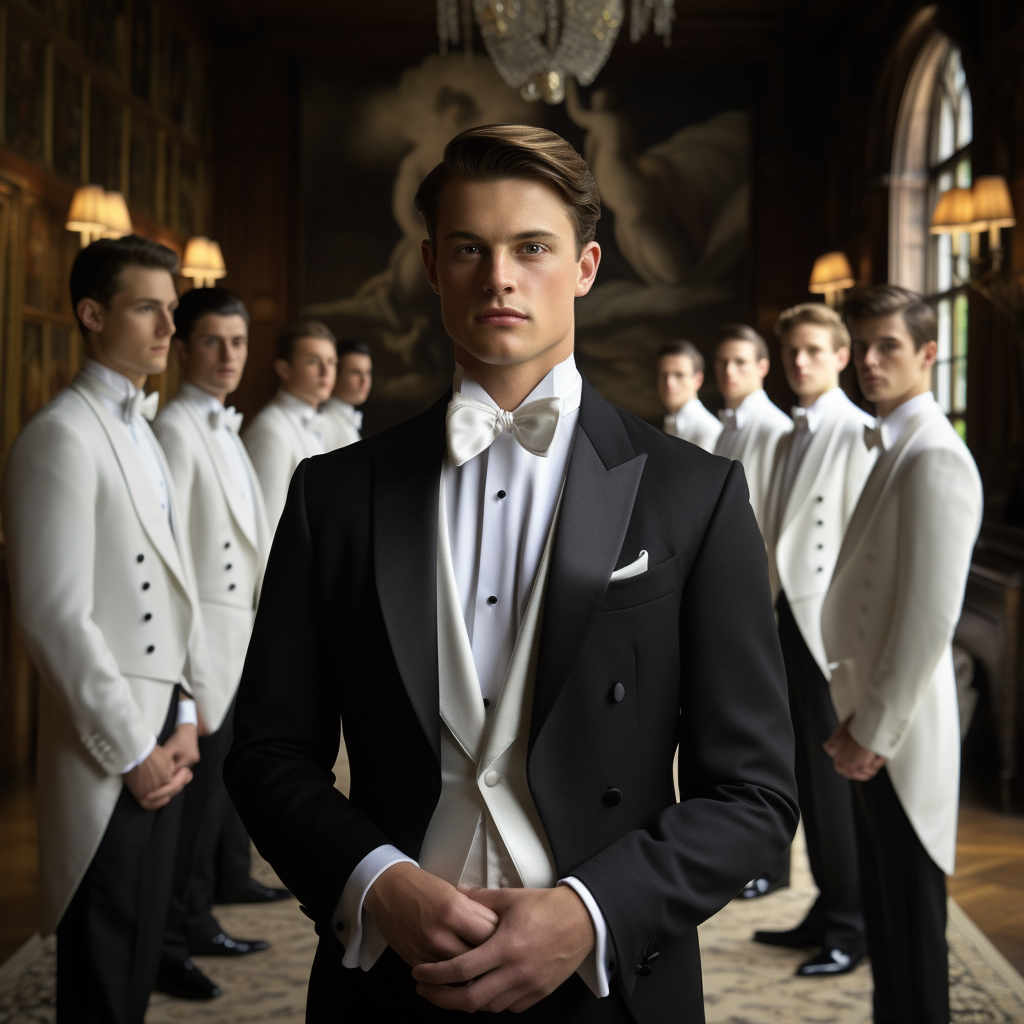This photograph captures a handsome, confident young Caucasian man in his late 20s, impeccably dressed for a formal event, likely a wedding. He stands prominently in the foreground, adorned in a dark tuxedo jacket with white vest, white bowtie, and a white shirt with cufflinks and buttons, accentuating his immaculate hair and well-groomed appearance. Flanking him are eight young men, presumed to be his groomsmen, each dressed in white tuxedos with white jackets, cummerbunds, and bowties. The group is positioned in a sophisticated hall, likely a formal dining room, replete with elegant sconces on the walls, a blurry chandelier above, a Persian rug underfoot, and a large, indistinct painting - possibly depicting angels - in the background. The overall ambiance suggests a grand and celebratory occasion.